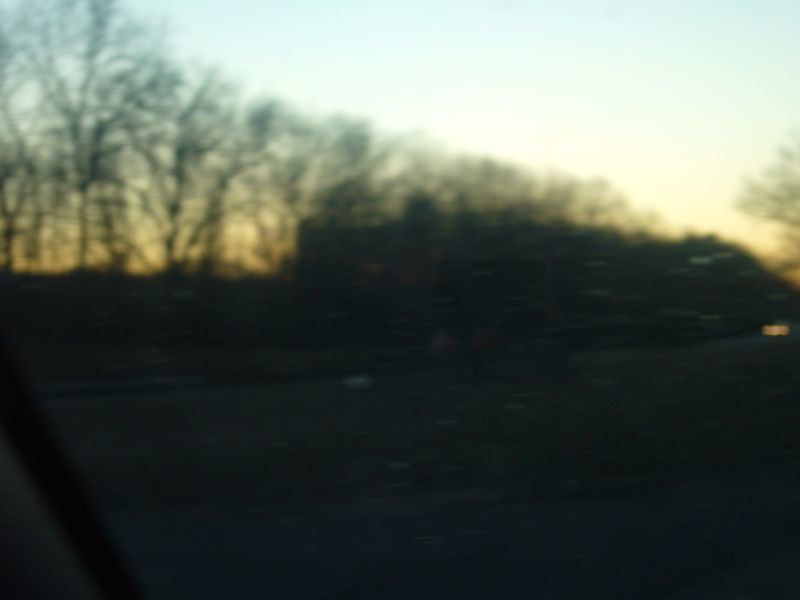In this evocative evening scene, the sun is on the cusp of setting, casting a muted light that hints at the transition from day to night. The season is likely fall, as suggested by the bare branches of a leafless tree silhouetted against the dimming sky. The photograph, snapped from the interior of a car, captures the atmosphere through the blur of an out-of-focus lens. Raindrops cling to the car window, creating a textured effect that adds depth to the image. Bright headlights from oncoming traffic pierce through the haze, illuminating the rural road flanked by numerous trees, including a set of evergreens that provide a striking contrast in their dark, green hues. Despite the lack of sharpness, the image conveys a palpable sense of tranquility and the quiet anticipation of an evening drive through the countryside.